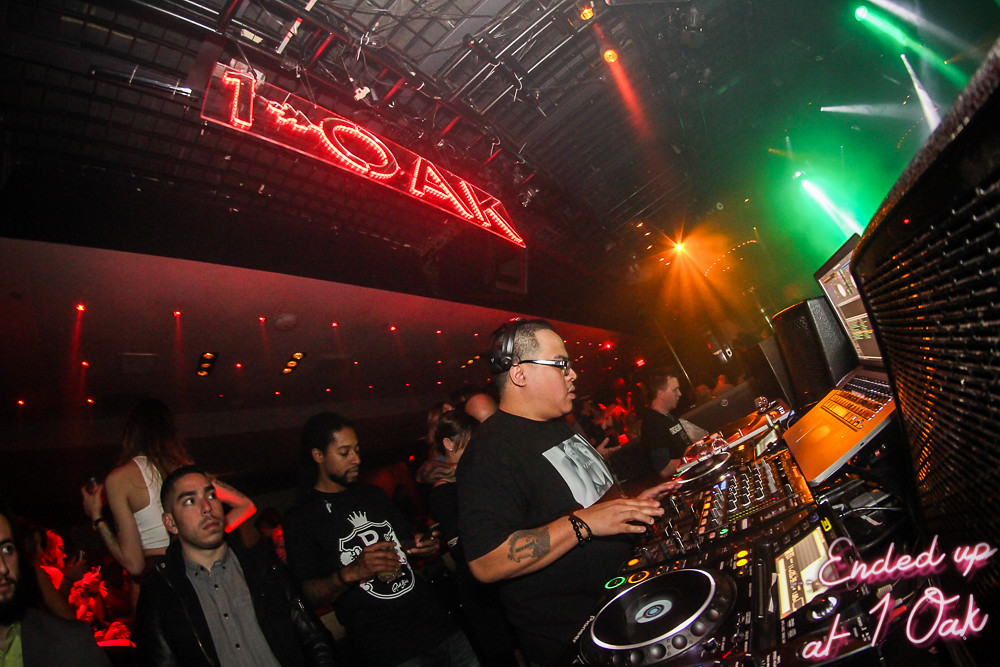The photograph captures the vibrant energy of a packed indoor party club DJ event, set in what appears to be a warehouse. The scene is drenched in a kaleidoscope of neon lights and signs, with prominent green, orange, and red hues illuminating the space. The focus is on two DJs performing at an impressively large DJ set, equipped with laptops, an array of knobs, turntables, and numerous vinyl records. The ceiling overhead reveals a network of pipes and wires, adding to the industrial feel of the venue.

A throng of people is both dancing and chilling behind the DJs, some engrossed in their phones while others hold drinks and socialize, clearly enjoying the lounge and bar area in the background. The photograph also captures a sense of urban sophistication with signage that reads "One Oak," and an inscription at the bottom right corner saying, "Ended up at One Oak," using the numeral '1' instead of the word "one."